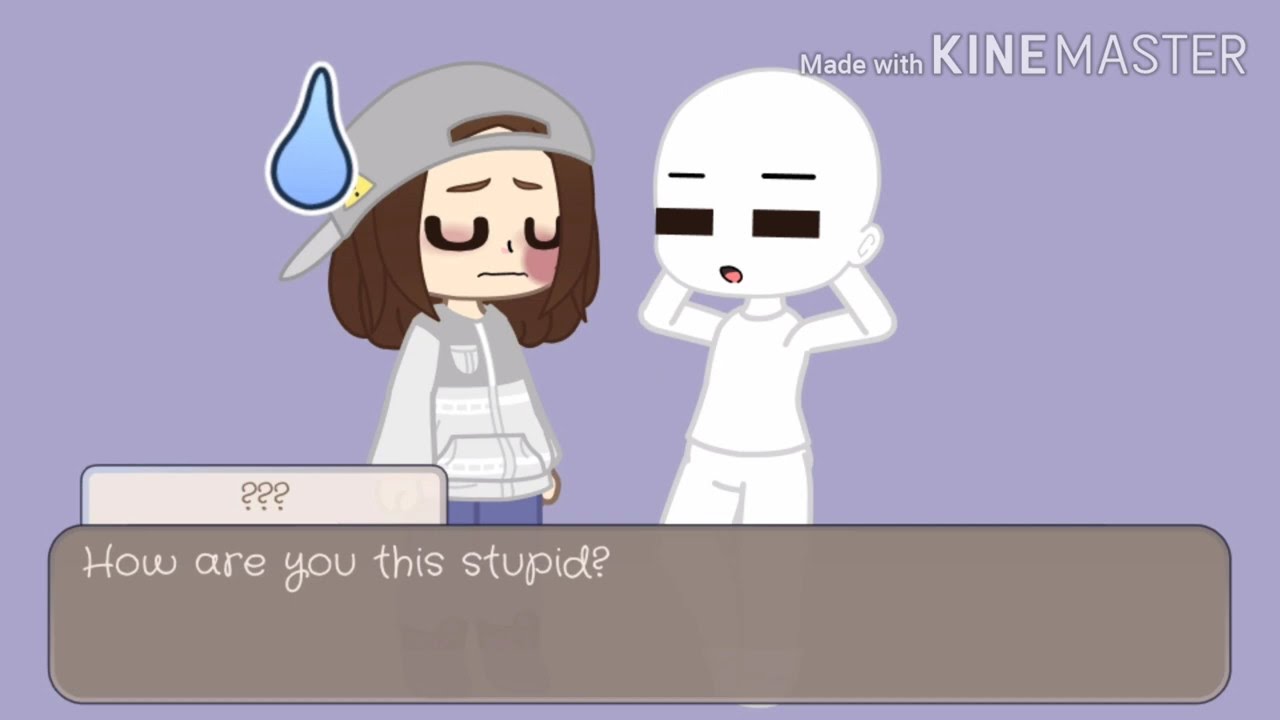In this detailed cartoon illustration set against a light purple, almost lavender background, the scene features two distinct characters engaged in conversation. On the left stands a girl with shoulder-length brown hair, a gray backwards baseball cap adorned with a small yellow symbol partly obscured by a blue teardrop, a gray hoodie with white pockets and sleeves, and blue jeans. Her eyes are closed, suggesting sadness, with a potential bruise or makeup around one eye and a thin, straight line for a mouth indicating distress. To her right is a ghostly white, bald character with solid black rectangular eyes and eyebrows, and a small oval mouth. The cartoon includes a grayish rectangular text box at the forefront with white cursive lettering that reads, "How are you this stupid?" A smaller white rectangle with three black question marks floats above. The top right corner of the image features a trademark notice, "Made with KineMaster," in uppercase letters.